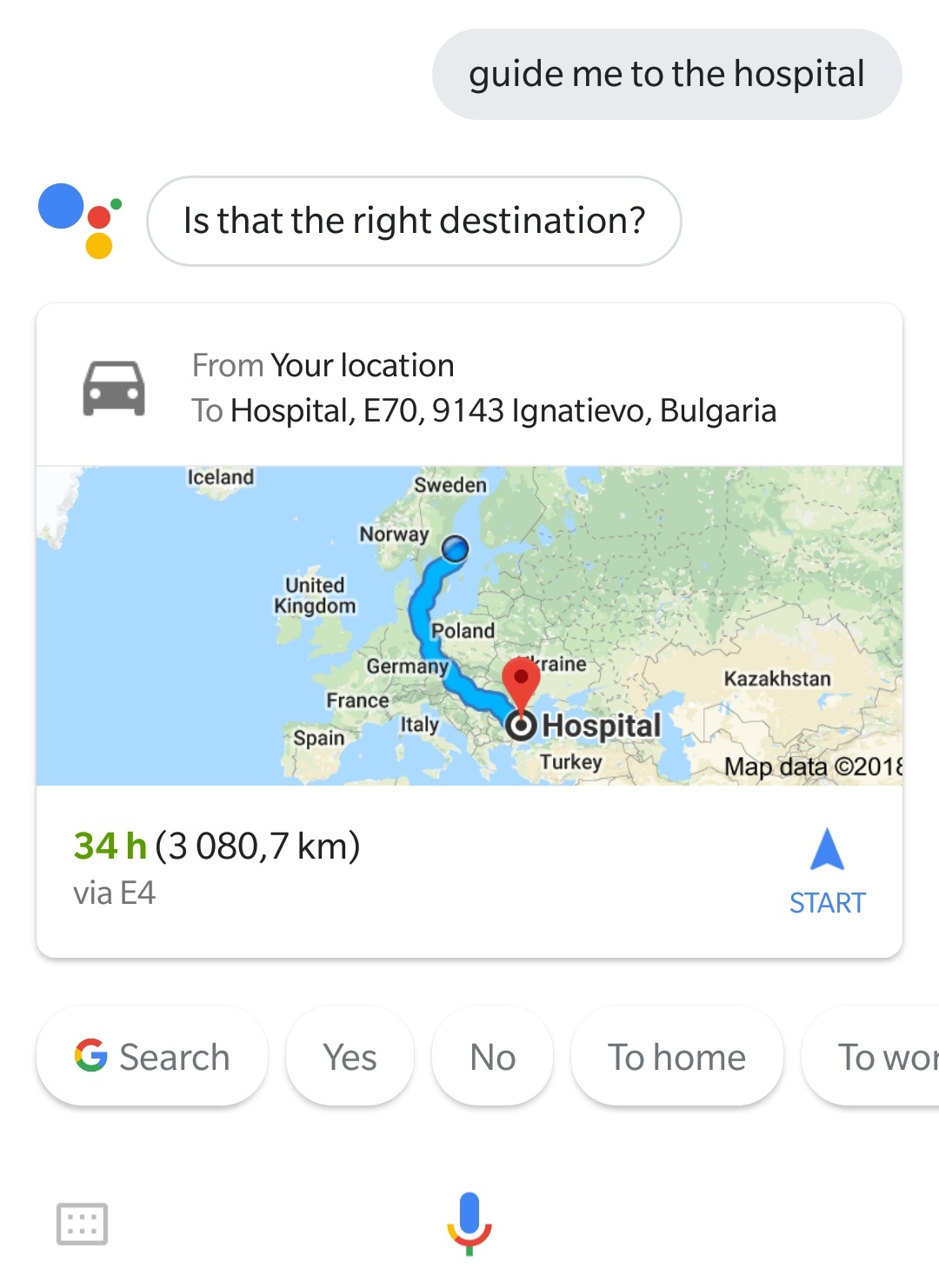A user in Sweden asks their AI assistant for directions to the nearest hospital. However, the AI, depicted with an avatar of four color-coded circles – a large blue circle, a slightly smaller red circle, a larger yellow circle, and a tiny green dot – misinterprets the request. Instead of finding a nearby hospital, the AI plots a course to a hospital in Nevestino, Bulgaria, a staggering 3,880.7 kilometers away. Displayed on the map, the route suggests a 34-hour drive via E4 and E70. This humorous error is highlighted by the onscreen options: "Yes," "No," "Home," or "Something else." The AI’s confusion between countries emphasizes the comical mishap in what should have been a straightforward task.